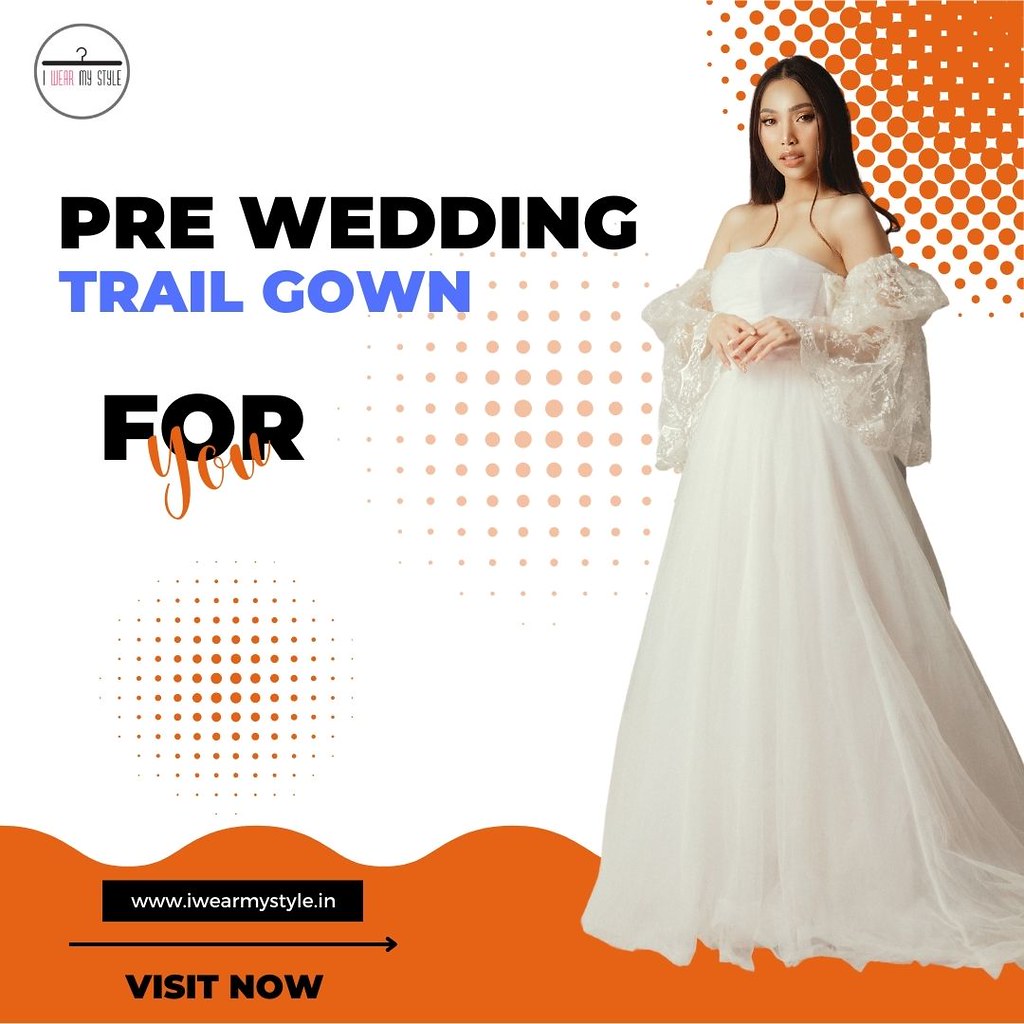This is a graphic advertisement for wedding gowns featuring a young Asian woman with long, straight black hair, standing on the right side in a long, flowing, strapless white gown. The gown has lace detailing around the dropped sleeves just below the shoulders, adding a delicate touch to its otherwise conservative yet elegant design. To the left of the woman, the text reads "Pre-Wedding Trail Gown For You", with "for you" highlighted in cursive orange letters. The graphic also includes an orange wavy design at the bottom, overlaid with a black box containing the URL "www.iwearmystyle.in" in white letters and a black arrow pointing to the right. Below this, bold black letters prompt viewers to "Visit Now". The entire advertisement is set against a clean white background, enhancing the gown’s pristine look.